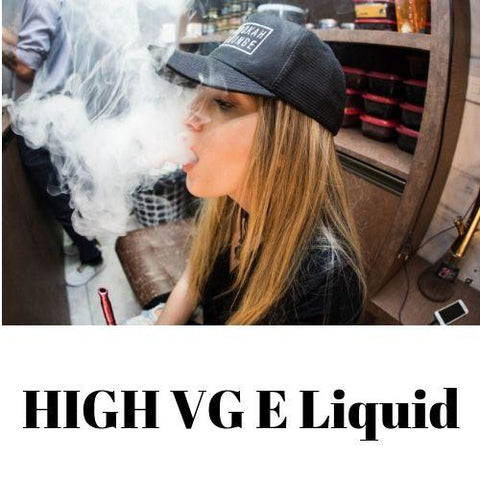In this advertisement for a vaping product, a young Caucasian woman with long, dirty blonde hair and dark streaks is featured. She is exhaling a large cloud of vape smoke that partially covers a man in the background. The image is taken with a fisheye lens, which warps and curves the sides. The woman is seated in a brown wooden chair and wears a black baseball cap with a white square displaying black text, and a black T-shirt. Her vaping pen is visible, held low with only the tip in view. The background includes shelves with red coverings arranged in rows, various items, and a partially visible laundry basket. Below the image, on a white background, the text reads "HIGH VGE LIQUID" in bold, capital letters. The overall scene suggests a promotional image for a vape shop, potentially used in social media campaigns.